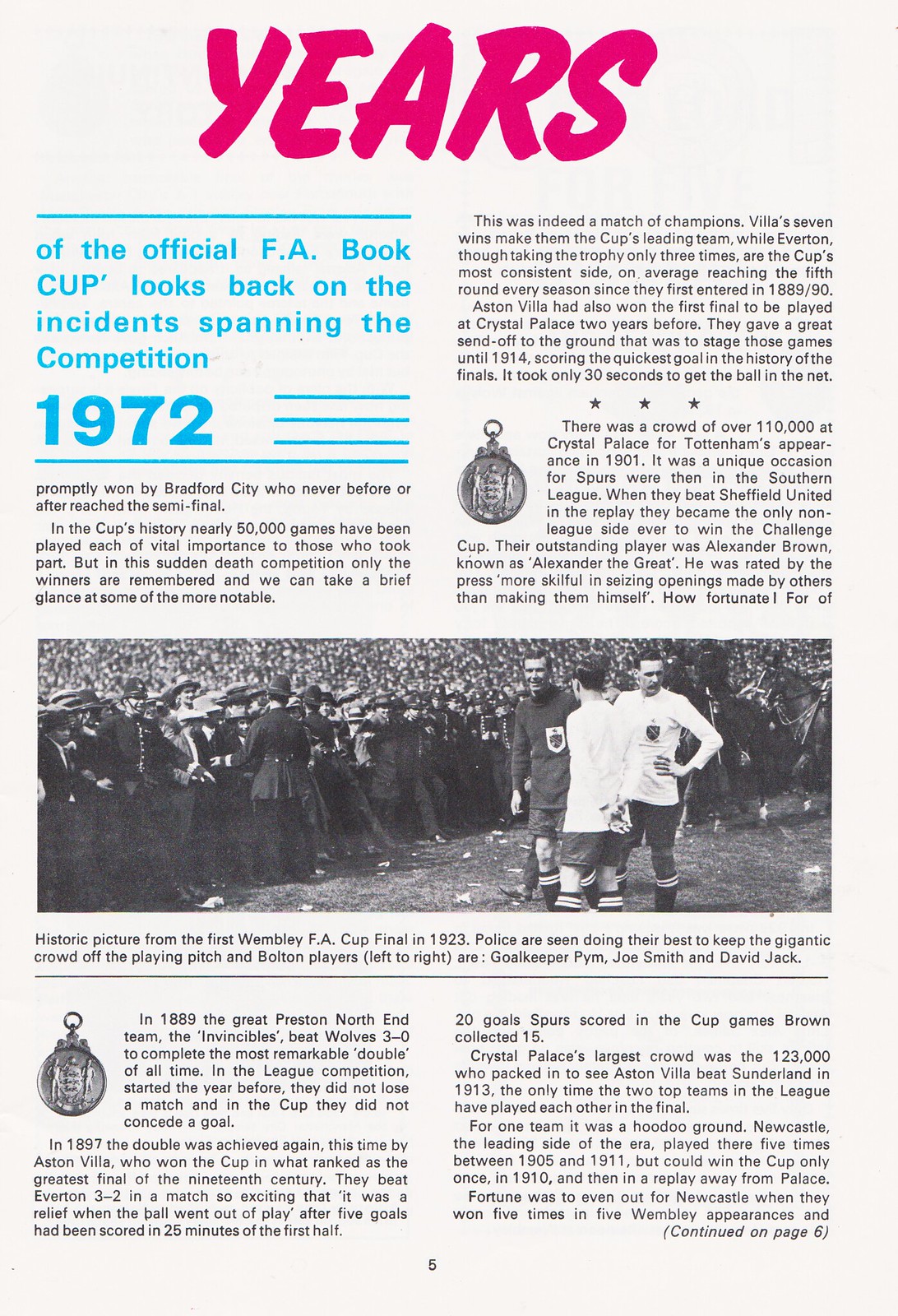This image depicts a page from an official game day program or magazine, specifically page number five. The page is a scanned copy featuring an article with magenta, cyan, and black inks. At the top, the word "YEARS" is prominently displayed in a unique magenta font, followed by a cyan pull quote: "of the official FA Book Cup looks back at the incidents spanning the competition 1972." The article includes two columns of small black text, intersected mid-page by a large photo from the first Wembley FA Cup final in 1923. The black-and-white image shows a massive crowd surrounding three soccer players—goalkeeper Pim, Joe Smith, and David Jack—while police strive to keep the crowd off the playing field.